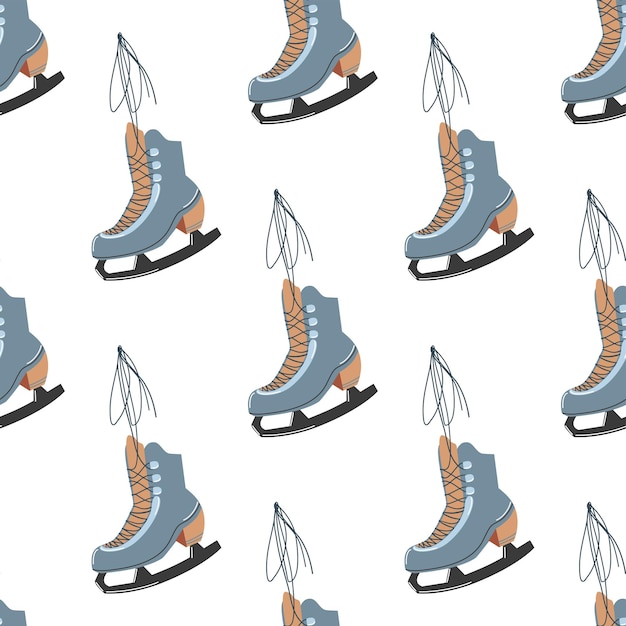The digitally-rendered image showcases a repeating pattern of ice skates on a white square background. Each ice skate features a predominantly grey body with very light grey, almost white accents. The heel and the tongue of the skate are both an orangish beige, while the inside of the skate, visible around the top edge, shares a similar orangish tone. The skates have black or dark grey laces that are drawn up beyond the top eyelets and hang down, appearing untied. The blade of each skate is black with a thin white line. This pattern is repeated multiple times, appearing approximately twelve times in total, though some skates are partially cut off at the edges. The skates are aligned diagonally from the bottom left to the top right, creating a uniform and visually intriguing design reminiscent of wallpaper or wrapping paper.